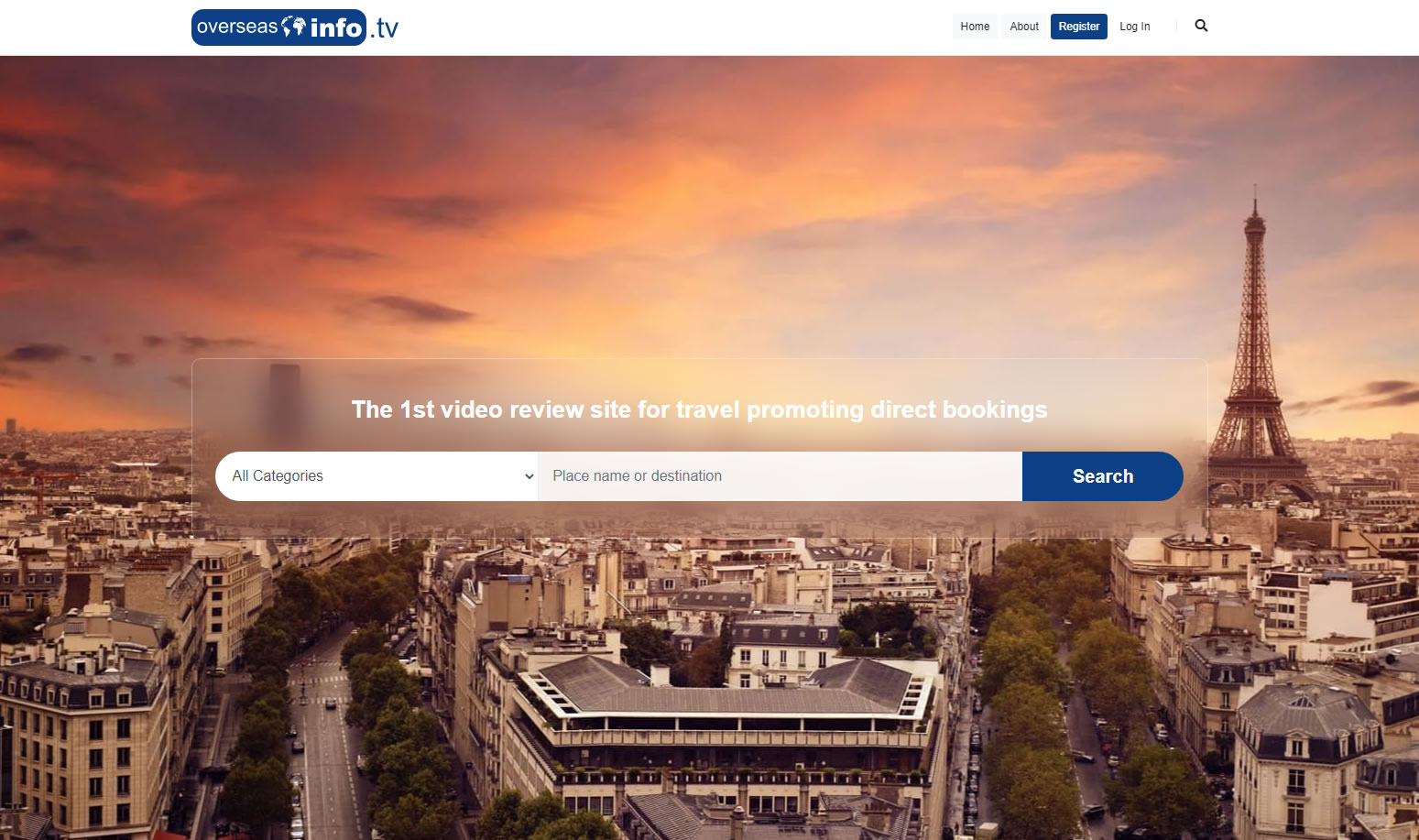The image showcases the homepage of a website dedicated to travel reviews and bookings. The background prominently features an aerial view of Paris, France, taken at dusk, with a beautiful pink sunset casting its glow mainly on the left side of the image. The iconic Eiffel Tower stands tall on the left side of the skyline, amidst a sprawling cityscape characterized by tree-lined streets and roads. 

At the top left of the website, there is a blue oval icon with white text that reads "overseas info" and includes a small image, followed by ".tv" outside the oval. On the right side of the header, there are four black buttons labeled "Home," "About," "Register," and "Login." The "Register" button is highlighted with a blue box and white font. Additionally, there is an image of a magnifying glass, indicating a search function.

In the center of the Paris image, a white, semi-transparent box contains blurred portions of the Paris skyline beneath white text stating, "The first video review site for travel promoting direct bookings." Within this box, there are two search fields: one for "All Categories" with a dropdown arrow, and another for "Place, Name or Destination," also with a dropdown arrow, followed by a "Search" button.

The overall design captures the essence of discovery and convenience, inviting users to explore travel opportunities through direct, video-based reviews.